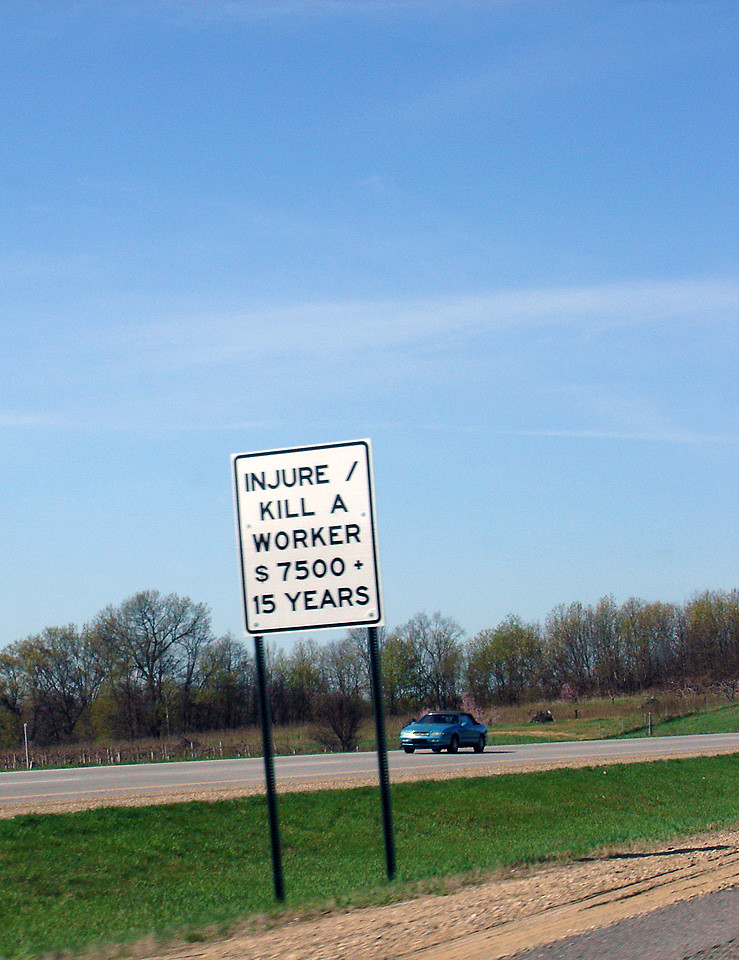The image depicts a rectangular, white road sign bordered by a black line, mounted on two vertical support bars. The sign is situated in the median of a roadway and bears a stern warning in black font: "Injure/Kill a Worker $7,500 + 15 Years". In the background, a blue car is approaching from the left side of the image, while beyond the roadway, a tree line is visible, adding a natural backdrop to the scene.